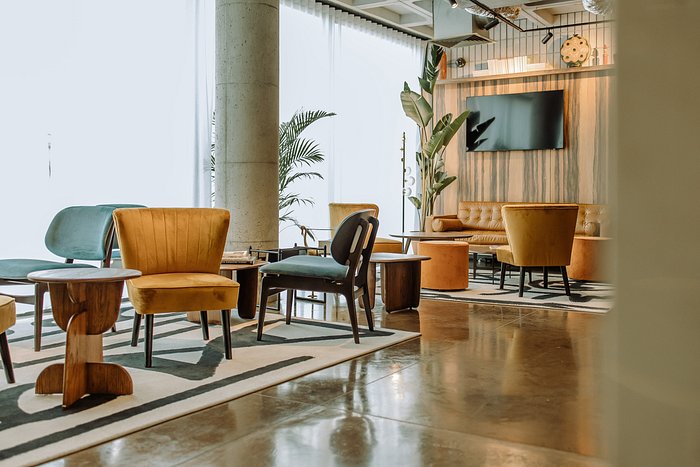The image depicts a modern lounge area or possibly a waiting room with contemporary interior design. A flat-screen TV is centrally mounted on the wall, with a shelf above it holding a mysterious white object and a circular art piece resembling a large coin or cookie. The background features two tropical decorative plants and a sturdy concrete column supporting the structure. The seating arrangements include a mix of light brown leather or pleather couches and chairs with green cushions, accompanied by wooden tables suitable for placing drinks. A white rug with a black line pattern lies on the shiny, stamped concrete floor, completing the sleek and polished look of the space.